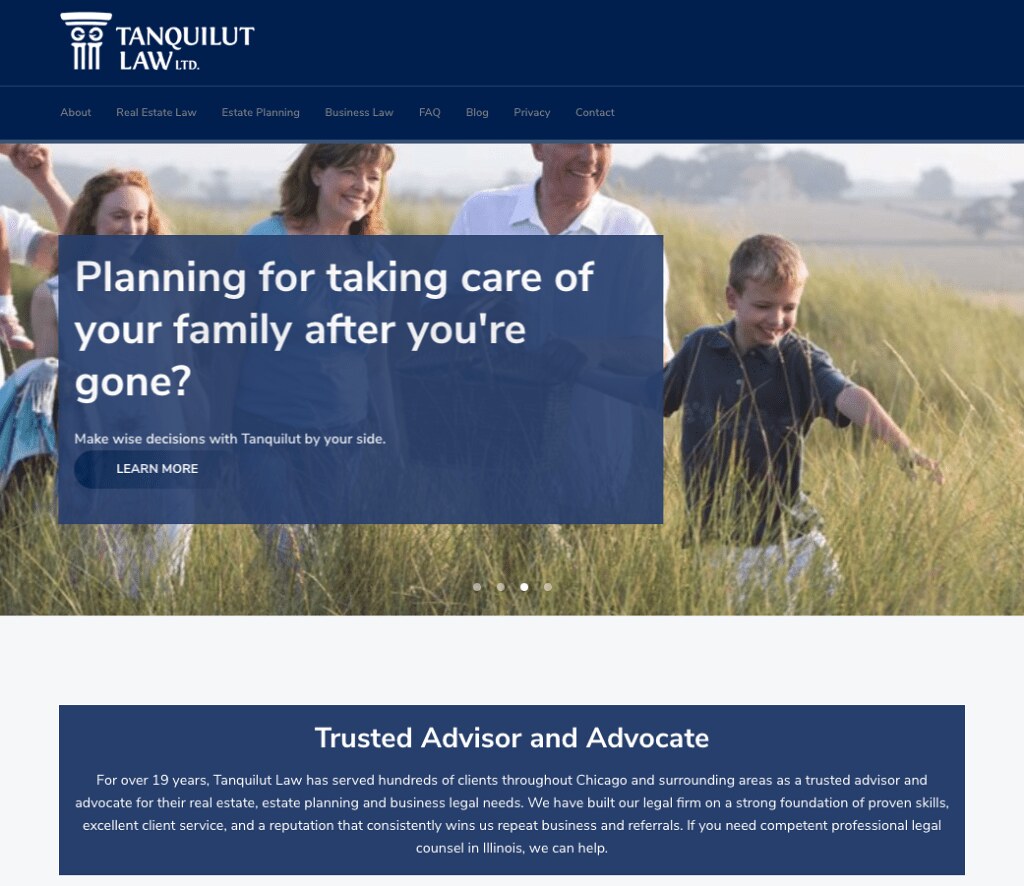This screenshot, likely taken from a website, features the header "Tanquillet Law, LTD." in white lettering against a blue background. A Greek pillar-like symbol is situated next to the text. Below the header, a navigation bar includes links to pages such as Real Estate Law, Estate Planning, Business Law, FAQ, Blog, Privacy, and Contact. The main section showcases a photo of a family of five walking through a long, grassy field, evoking a countryside or farm setting. The family, composed of a father, mother, son, daughter, and another relative, is dressed in casual attire like t-shirts and button-down shirts. A semi-transparent blue box overlays the image, displaying the message in white text: "Planning for taking care of your family after you're gone. Make wise decisions with Tanquillet by your side." Below, in deeper blue, there's a clickable oval labeled "Learn more." Further down, the text shifts to white again, reading, "Trusted advisor and advocate," followed by information about the firm's history, including its long-standing presence in Chicago. The overall color scheme includes shades of blue, off-green, white, brown, and gray.